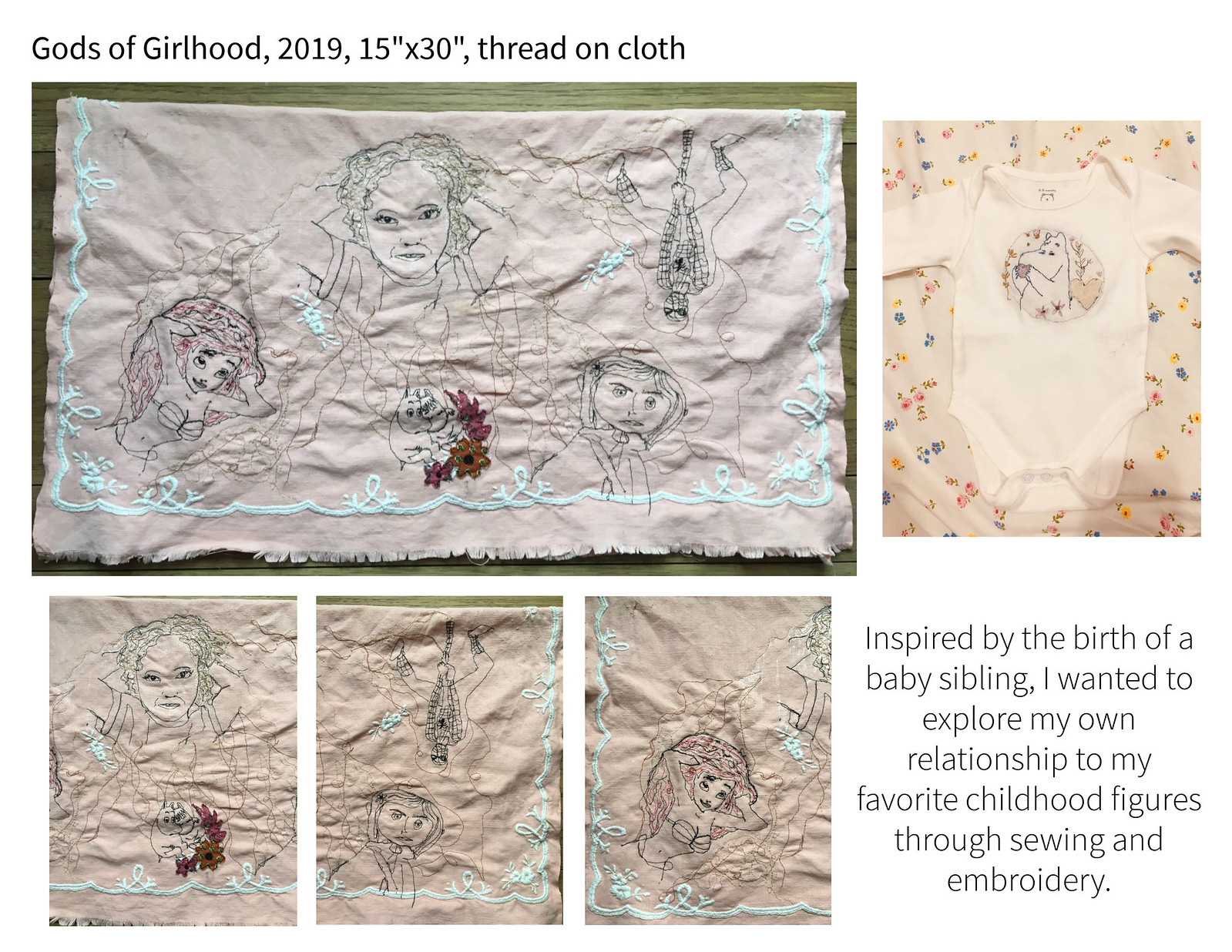The image showcases a collection of embroidery work set against a white background. Dominating the display, a large embroidered handkerchief occupies approximately two-thirds of the upper left corner, adorned with intricately embroidered cartoon characters including Ariel, the mermaid, Coraline, Moomin, an elderly woman, and Spider-Man, all surrounded by light blue floral border designs. Below the large piece are three smaller embroidery pieces. On the right side of the image, there is another lengthy embroidery piece, nearly the same height as the large one on the left. In the bottom right corner, a legless baby onesie features a finely embroidered image of Moomin. Black text captions anchor the image, with the top reading, "Gods of Girlhood, 2019, 15 inch by 30 inch, thread on cloth," and the bottom right providing context with, "Inspired by the birth of a baby sibling, I wanted to explore my own relationship to my favorite childhood figures through sewing and embroidery."